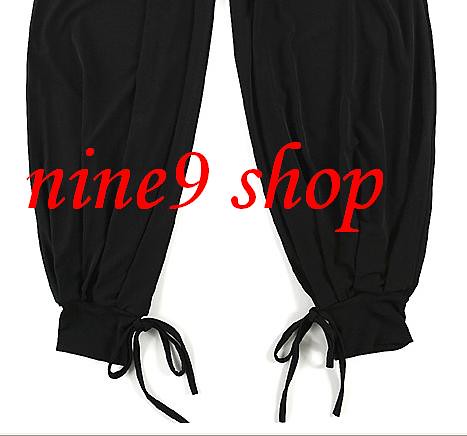The image depicts the bottom half of a pair of black jogging pants against a completely white background. The pants feature a lace detailing at each ankle, allowing them to be tied tightly. Above the pants, in italicized red font, are the words "NINE 9 SHOP," with "NINE" spelled out and the number "9" following it. The imagery focuses solely on the pants, emphasizing their unique design elements with no other elements in the frame. This minimalist presentation suggests it’s an advertisement for a product from a store called Nine 9 Shop, showcasing these distinctive jogging pants.